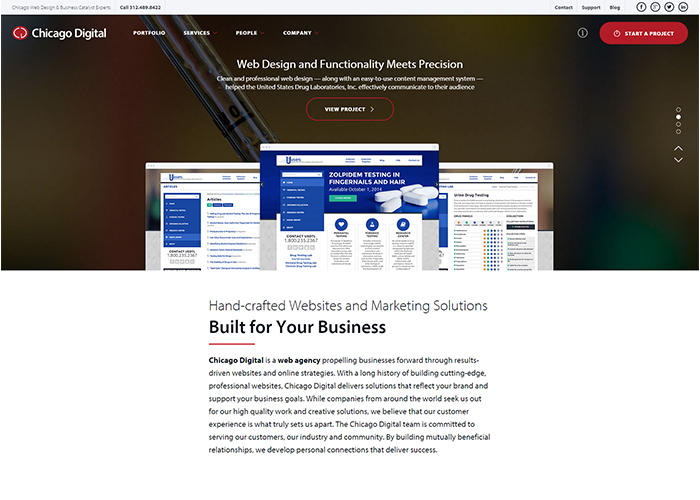Homepage of the Chicago Digital Website:

The homepage of the Chicago Digital website prominently features the company’s logo, followed by a navigational menu with tabs for Portfolio, Services, People, and Community. Each of these tabs is accompanied by a red drop-down arrow. At the very top of the page, a light gray banner displays a phone number in black text, accompanied by options for Contact and Support, as well as links to the Blog. Social media icons for Facebook, Twitter, LinkedIn, and another unidentified platform are also visible.

The main body of the page includes a central image, slightly out of focus, which appears to resemble either a computer or smartphone screen. Overlaying this image, bold text announces: "Web design and functionality meets precision," followed by smaller, unreadable subtext. Below this, an oval button labeled "View Project" invites user interaction.

Further down the page, three smaller screens pop up, predominantly showcasing blue and white designs. The middle screen displays the title "Zolpidem testing in fingernails and hair." Continuing, an article section headlines: "Handcrafted websites and marketing solutions," with a subtitle: "Built for your business."

The detailed content describes Chicago Digital as a "web agency propelling businesses forward through results-driven website and online strategies." With a long history of building cutting-edge professional websites, Chicago Digital delivers solutions that reflect a brand and support business goals. The company works with global clients, who seek out Chicago Digital for high-quality work and creative solutions. Emphasizing their commitment to customer experience, the Chicago Digital team is dedicated to serving customers, industry, and community by building mutually beneficial relationships and fostering personal connections that drive success.